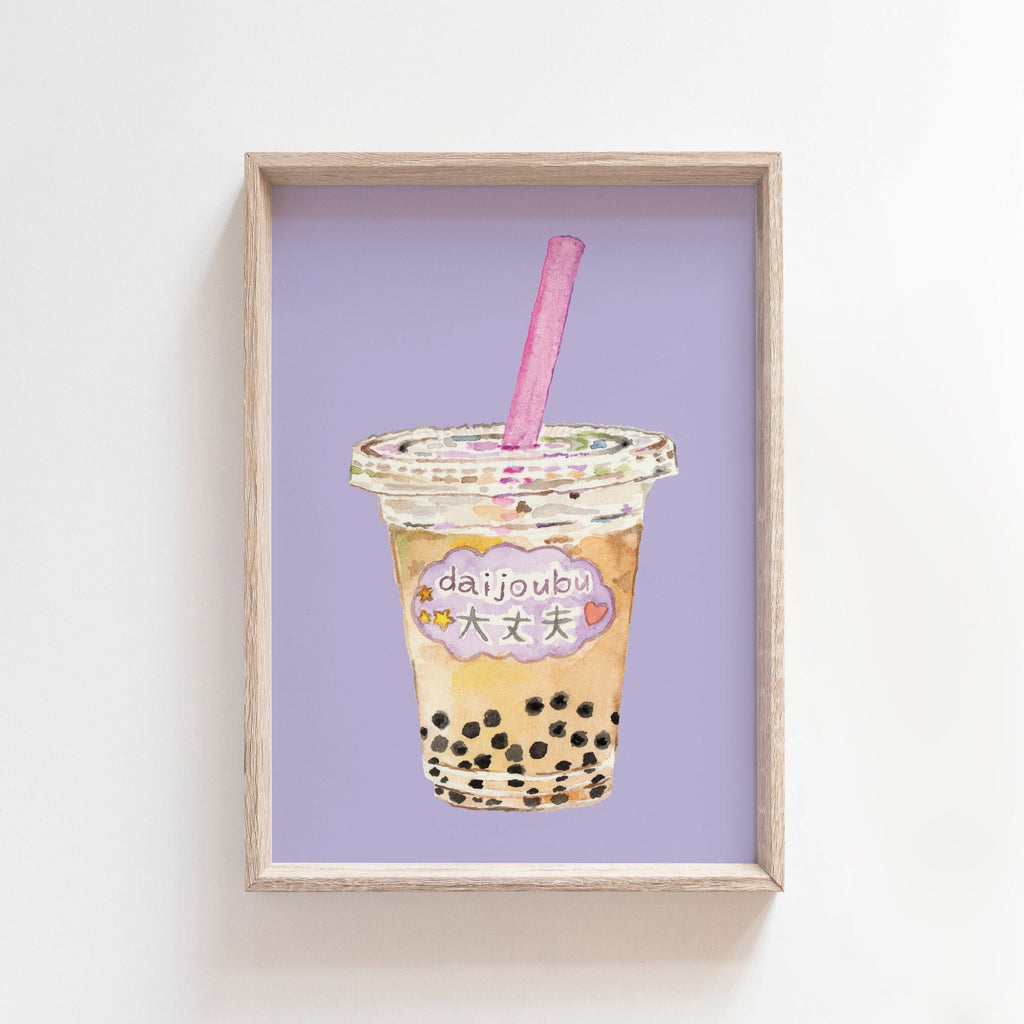This image depicts a detailed artwork hanging on an eggshell gray wall. The artwork is framed in a light blonde wood, giving it a subtle depth that enhances its box-like presentation. Inside the frame, there is a vibrant illustration set against a light lavender background. The centerpiece of the illustration is a plastic cup filled to the brim with a light tan boba milk tea. At the bottom of the cup, numerous black boba pearls are distinctly visible. The cup features a large, thick pink straw protruding from its plastic lid. Prominently displayed on the front of the cup is a cloud-shaped label that reads "Daijubu" in black text, accompanied by Japanese writing. This label is adorned with a small heart illustration and three stars colored yellow, orange, and red, which add a playful touch. The overall composition is bright and inviting, with subtle rainbow reflections on the cup and label that further enhance the visual appeal.